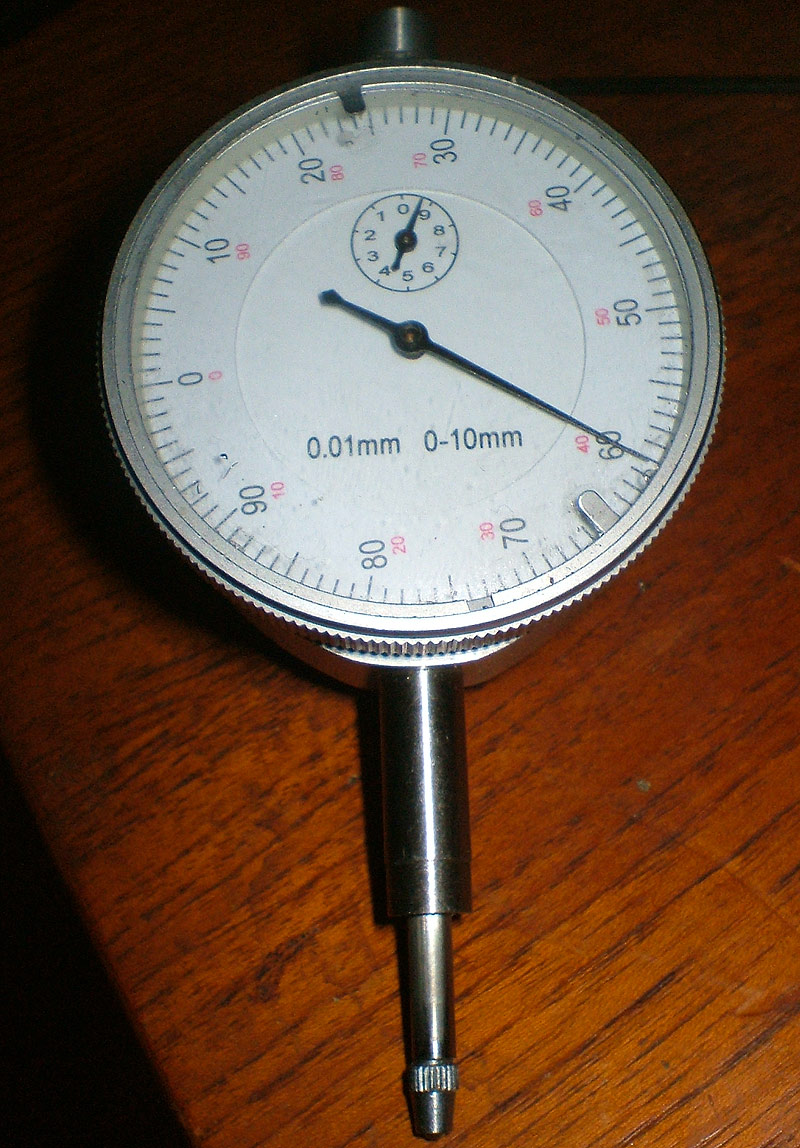This image features a precise measuring instrument that appears to be a pressure gauge or a specialized dial indicator rather than a thermometer. The device has a white face marked with numerical increments ranging from 0 to 90 along its outer edge. Dominating the center of the face is a secondary set of measurements, ranging from 0.01 mm to 10 mm, indicating highly detailed readings. The gauge only has a single hand, reminiscent of a second hand on a clock, suggesting that it measures continuous variables like pressure or displacement.

Supporting the gauge is a prominent handle or a pointed fixture extending from its base, the exact function of which is unclear. The device rests on a surface that is clearly a wooden table, with a distinct, natural grain pattern.

Additionally, the gauge’s face features a smaller inset dial with numbers running counterclockwise from 0 at the top to 9. This small clock-like feature is embedded within the primary measuring scale, adding another layer of detail to the instrument's functionality.